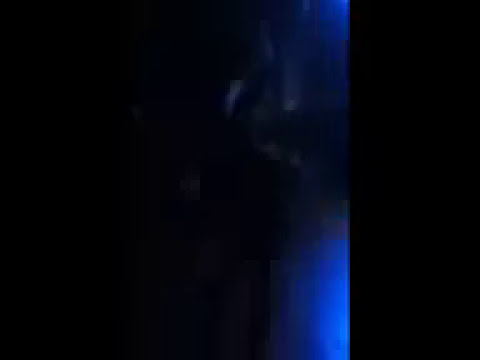This enigmatic image features a predominantly dark composition, shrouded in mystery with varying degrees of blackness and blue lighting. The right quarter of the square photo is a solid black stripe, contrasting sharply with the adjacent blue streak occupying the next 25%. This blue streak, darker in the center and brighter at the bottom, transitions seamlessly into the surrounding black, giving an eerie, haunting vibe. The left side of the image is a mix of hazy blacks and grays, suggesting something amorphous is emerging from the shadows. The top right corner also contains subtle hints of blue, adding to the spectral atmosphere. Jagged, fang-like shapes protrude within the blue area, further enhancing the ghostly and menacing feel of the scene. The overall impression is that of an abstract, possibly artistic depiction of a ghostly apparition in a dark, underwater setting.